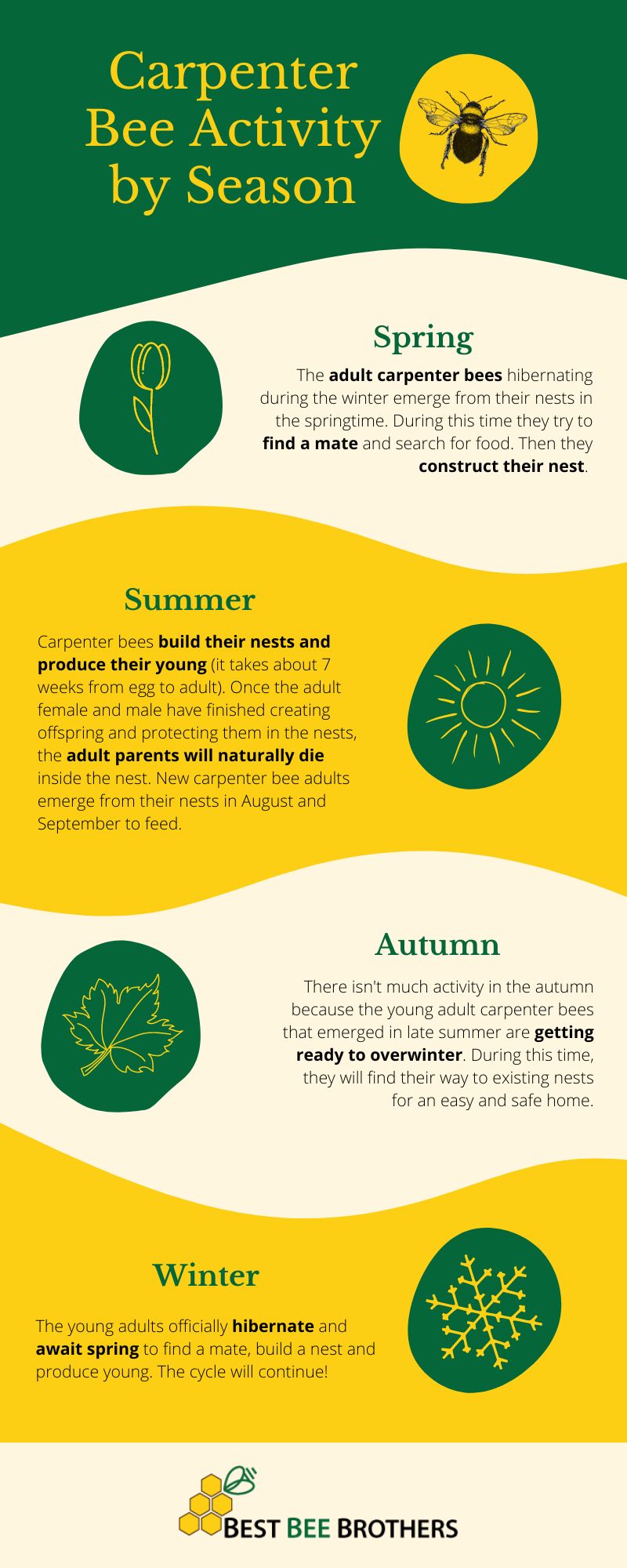The infographic, designed in an elongated vertical format, details "Carpenter Bee Activity by Season" at the top in yellow text against a green backdrop. Below, a yellow circle featuring a black and yellow striped carpenter bee illustration is present. The layout is divided into four curving sections representing spring, summer, autumn, and winter, each distinguished by alternating off-white and yellow backgrounds. Within each section, green lettering names the season, accompanied by green circles with yellow seasonal icons: a flower for spring, a sun for summer, a leaf for autumn, and a snowflake for winter.

In the spring segment, the off-white background features a description of adult carpenter bees emerging from hibernation to find mates and food, followed by nest construction. The summer section, on a yellow background, describes the bees building nests and producing offspring, detailing the seven-week period from egg to adult, and notes the natural death of adult carpenter bees after this process. Autumn, back to off-white, explains the minimal bee activity as young adults prepare for winter by finding existing nests. The winter portion, set against a yellow background, states that young adults hibernate until spring, continuing the cycle.

The bottom section contained within a tan border highlights the text "Best Bee Brothers," indicating the infographic's creators.